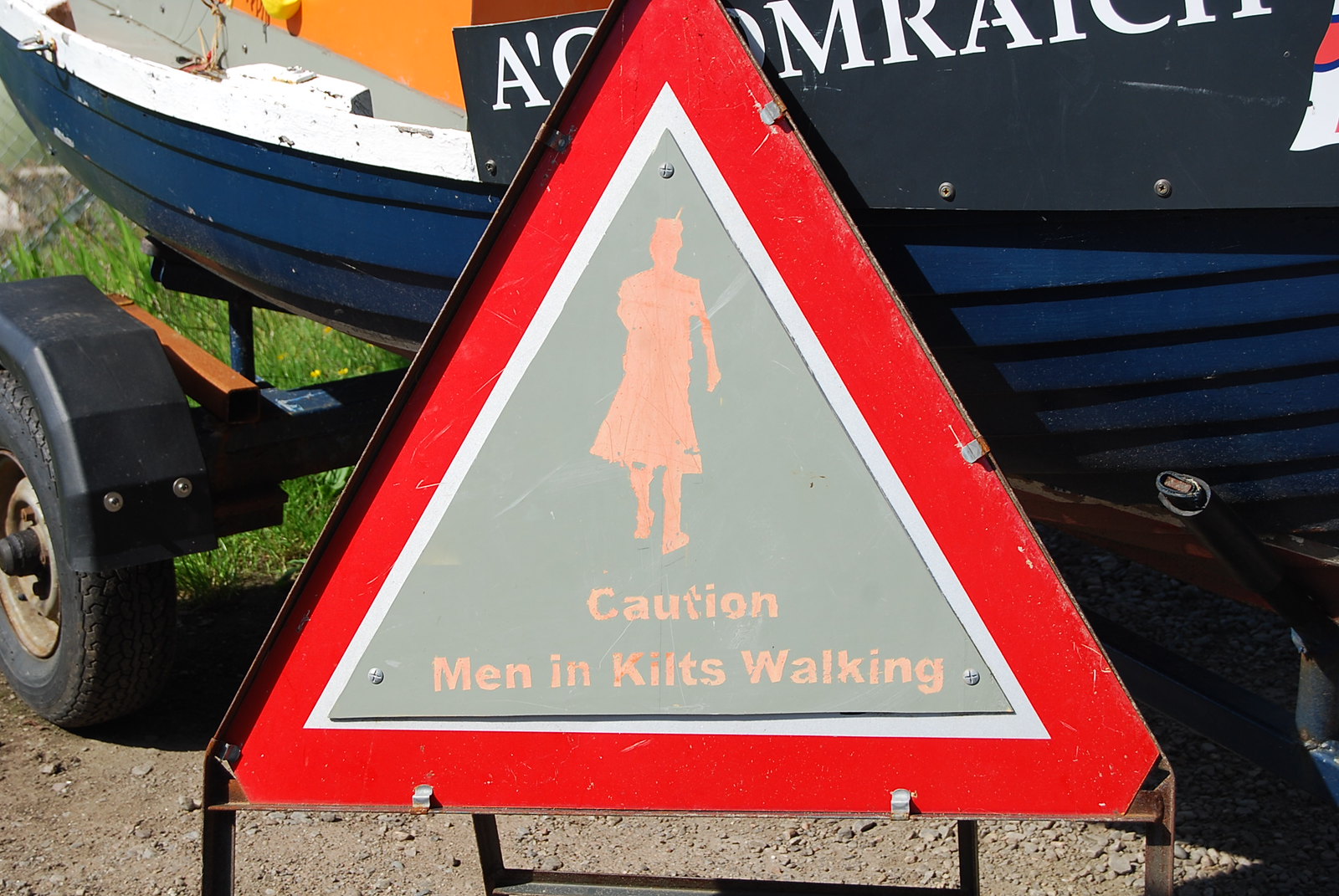The photograph depicts a metal warning sign shaped like a triangle with a red border and a grey interior. At the center of the triangle is a peach-colored silhouette of a person wearing a kilt, accompanied by the text "Caution: Men in kilts walking," also in peach. Behind the sign, there is a partial view of a blue and white boat mounted on a trailer, with the boat displaying some partially visible writing. The background includes a grey floor and a patch of green grass, enhancing the scene's outdoor setting.